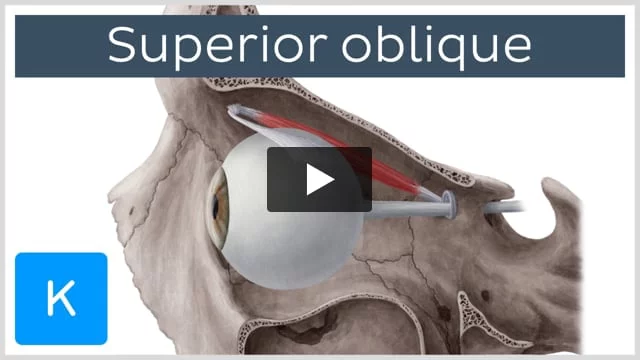The image appears to be a screenshot from a video interface, likely taken from a web page. It is a horizontal rectangle outlined with a thin gray border. Across the top of the image is a dark gray band featuring the words "Superior Oblique" in white text. Prominently in the center, there is a gray rectangle with a white arrow pointing to the right, resembling a play button. The detailed background of the image shows an anatomical diagram of an eye and its surrounding structures. The eye is positioned somewhat centrally and is depicted with a white sclera and a brown iris, appearing to look towards the left. Behind the play button, you can observe the eye's anatomical components: a white rod extends back through an opening, while another white rod with red accents connects above the eye. To the right of the eye are parts of the skull, illustrated with brownish tones, anchoring the eye in its socket. In the bottom left corner of the image is a blue square containing a white letter "K".